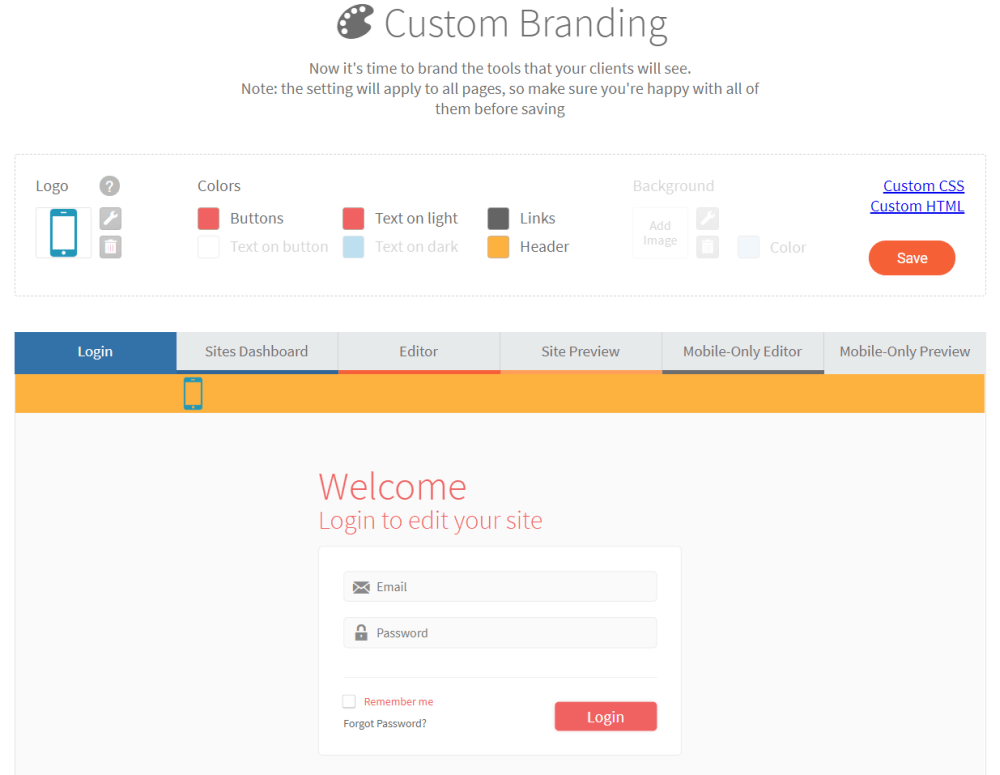The image is a detailed screenshot of a website's login page with a focus on custom branding features. The page has a light theme overall. At the top, a painter's palette icon in gray is prominently displayed next to the text "Custom Branding" also in gray. Directly below this, in smaller and lighter gray text, there is an instructional note: "Now it's time to brand the tools that your clients will see. Note, this setting will apply to all pages, so make sure you're happy with all of them before saving."

Below this text, there is a long rectangular box with a white background. On the far left of this box, the word "Logo" is written. Adjacent to this, there is an icon depicting the front view of a cell phone screen with icons for a wrench, a garbage can, and a question mark button next to it. 

Further down, there are additional selection boxes labeled "Colors," allowing users to customize the colors of buttons, text, links, and headers. Towards the far right of the rectangular box, a prominent red button with white text reading "Save" is visible.

Below these elements, there are multiple navigation tabs, with the "Login" tab currently selected. The lower part of the page features a large area with a white background, housing a white login box where users are prompted to enter their email and password.